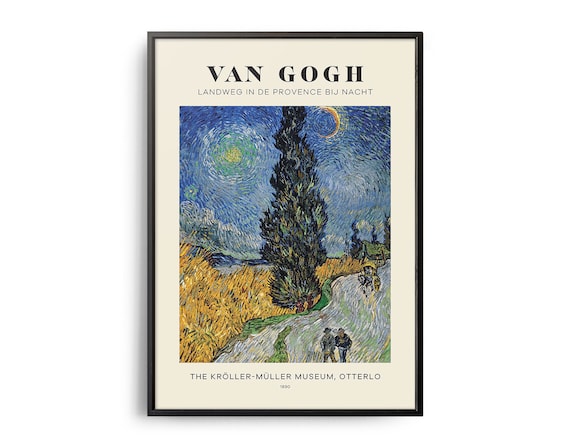This detailed image is a reproduction of Vincent Van Gogh's painting titled "Road with Cypress and Star," presented within a black frame. The artwork itself is mounted on a white backing. At the top of the display, "Van Gogh" is prominently displayed in bold black letters. Just below, in smaller black letters, is the text "Landweg en de Provence bij nacht." Beneath this text lies the evocative painting.

The scene features a tranquil night with a small crescent moon and a star set against a deep blue sky, embodying Van Gogh's characteristic textured, wavy design. Dominating the background are golden yellow fields, adding warmth to the composition. A towering cypress tree stretches from the road up through the center of the image. In the foreground, the winding road leads two figures, presumably walking together, towards the horizon. The landscape includes brown wheat and green grass, suggesting a rural setting.

Below the painting, in smaller black letters, the institution is credited as the Kroller-Muller Museum in Otterlo. A date is also mentioned, though it is unclear and not fully visible.

Overall, this framed depiction captures the essence of Van Gogh’s masterful use of color and texture to convey a serene night scene in the countryside, harmoniously blending natural elements and human presence.